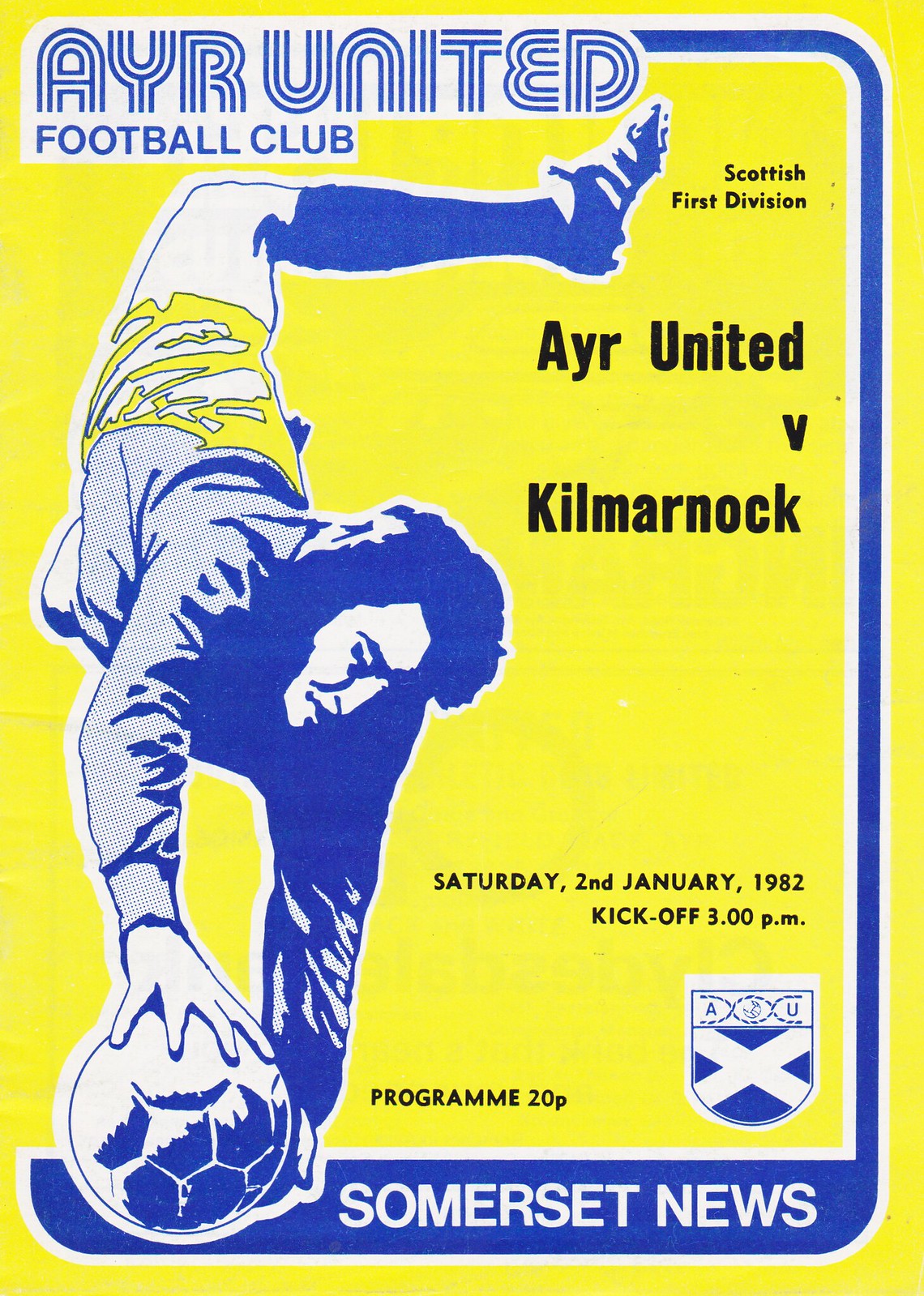This vintage poster from AYR United Football Club, Scottish First Division, features a dynamic image of a soccer player mid-action, seemingly performing a dramatic somersault with his left leg up in the air and his hand reaching toward a blue soccer ball. The player's dark blue shirt and yellow shorts are vividly highlighted against the predominantly lemon-yellow background. His fuzzy hair and light-skinned face are discernible in the blue-toned image. The poster is bordered on the right side by a blue stripe, with green and red lettering at the top that reads "AYR United Football Club." Important match details are prominently displayed: "AYR United versus Kilmarnock" in blue letters, followed by "Saturday, 2nd January 1982, kickoff 3 p.m." near the bottom. Additionally, "Program 20p" is printed centrally towards the bottom, and the banner at the very bottom reads "Somerset News" in white uppercase letters against a blue background.